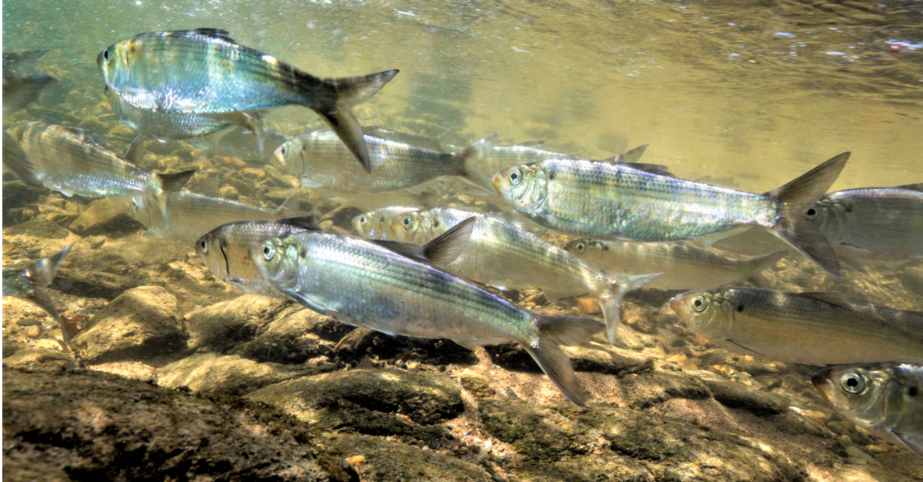This photograph captures an underwater scene in a shallow body of water, likely a stream or near a shoreline. The central focus is a school of small, narrow fish, possibly minnows, swimming from right to left. These fish are predominantly silvery with iridescent scales that shimmer in hues of green, blue, yellow, and white under the sunlight filtering through the clear water. Their tails are darker, appearing in shades of dark gray or silver, with distinctive black irises. The water is shallow enough, approximately a foot deep, that both the bottom and the surface are visible. Below the fish, the riverbed is composed of eroded rocks and boulders in various shades of tan, green, brown, and yellow, giving a textured and colorful backdrop to the scene. Above the fish, the top of the water surface can be seen, with light reflections mirroring the tones of the rocks below. The sunlight permeating the water adds a dimension of clarity and depth, making the harmonious movement of the fish the striking focus of the image.